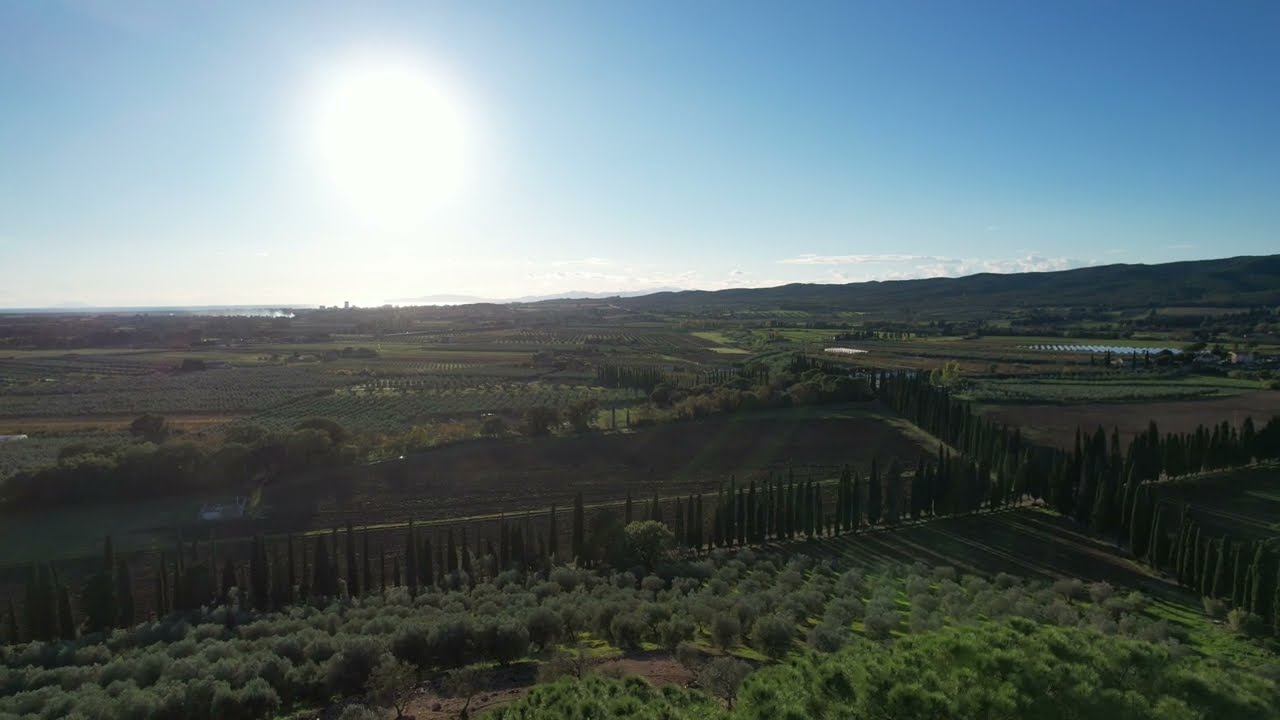The aerial photo captures a lush, green valley of farmland suffused with vibrant life. Numerous plots, each demarcated and brimming with diverse trees, plants, bushes, and hedges, stretch across the landscape. Some plots feature bright green trees of varying heights, while others remain fallow, their dark brown dirt freshly plowed. An assortment of tall and short, bushy and thin bushes adorn the land. Tall, skinny, dark green arbofites form an X-like pattern, dividing the farmland and lining a stone fence. In the foreground, verdant orchards, meticulously sectioned-off fields, and farm buildings are clearly visible. The backdrop reveals rolling green hills and distant mountains merging seamlessly with the horizon, above which the bright blue sky hosts a shining white sun. A slight reflection from the aircraft window hints at the elevated vantage point from which the photo was taken.